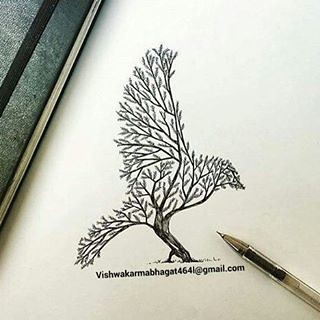The image depicts a simple yet intricate line drawing on a piece of paper. The sketch showcases a tree cleverly shaped like a bird. The tree's branches, all very straight and small, form the bird's features: the beak on the left, wings on the right, and the tail also on the left. The tree is curving away from the viewer, adding a dynamic aspect to the composition. In the upper left-hand corner of the image, a notebook is partially visible. Below the sketch, there are some barely legible words that seem to include the name "Vishnarak" and an email address ending in "@gmail.com." A pen with black ink rests on the paper, suggesting that the drawing was freshly completed.